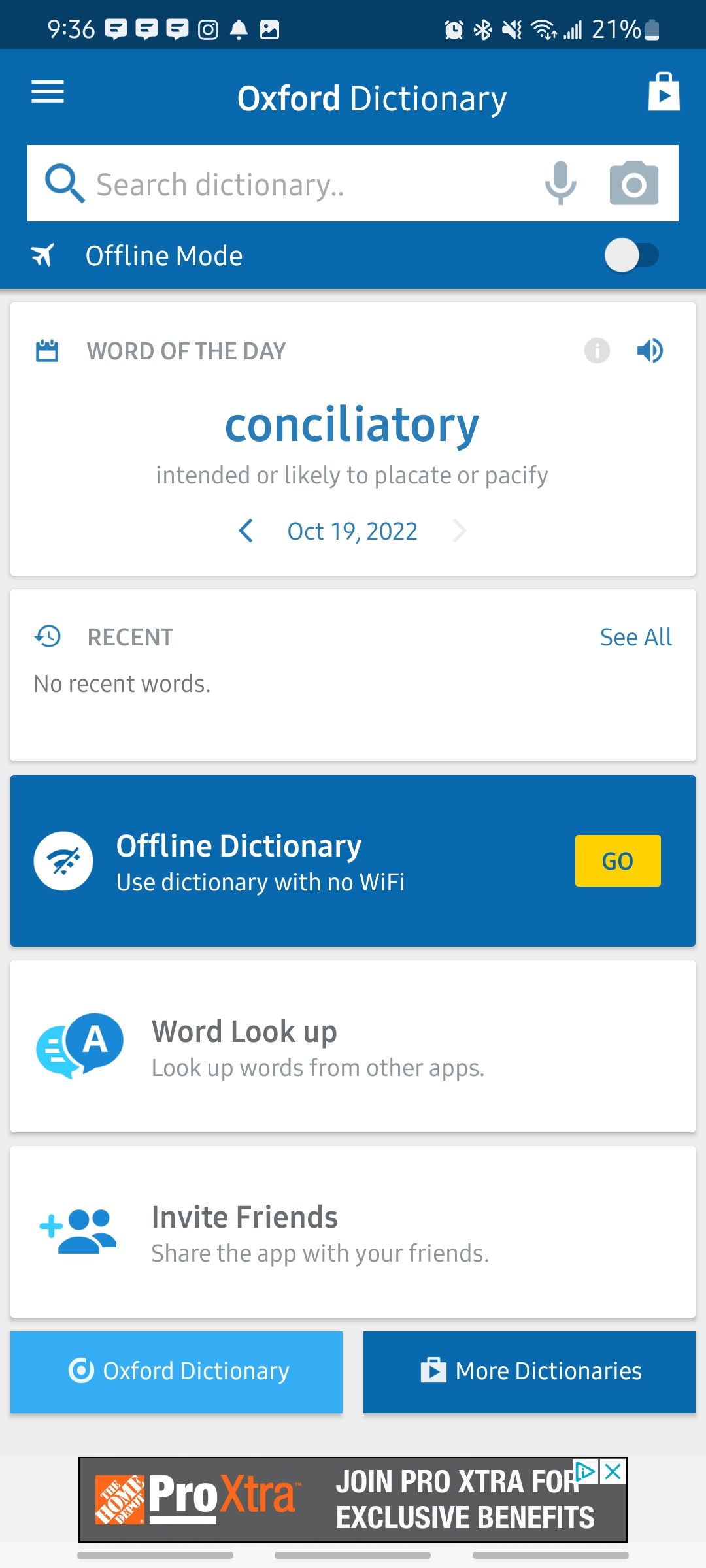This screenshot captures the interface of the Oxford Dictionary's website. At the top, a blue navigation bar prominently displays "Oxford Dictionary" in the center. On the left side of this bar, there is a three-bar menu icon, while on the right, a bag icon with a play button is visible.

Beneath this navigation bar is a search bar with the placeholder text "Search Dictionary." On the right end of the search bar, there are grey microphone and camera icons, indicating voice and visual search functionality, respectively.

Further down, still within the blue section, there is a label for "Offline Mode" accompanied by an airplane icon on the left. To the right of this label, there is a white toggle button.

Below the blue section, the interface is segmented into various white boxes. The top box is designated for "Word of the Day" and features the word "Conciliatory" in bold blue text in the middle. Beneath this, the definition "Intended or likely to placate or pacify" is provided in grey text. An accompanying blue back arrow, along with the date "October 19th, 2022," is situated right below the definition.

Further down, another white box titled "Recent" includes a "C all" link on the right side, suggesting a prompt to see all recent words. However, it currently states "No Recent Words."

The layout is clean and organized, reflecting the functionalities and features available on the Oxford Dictionary website.